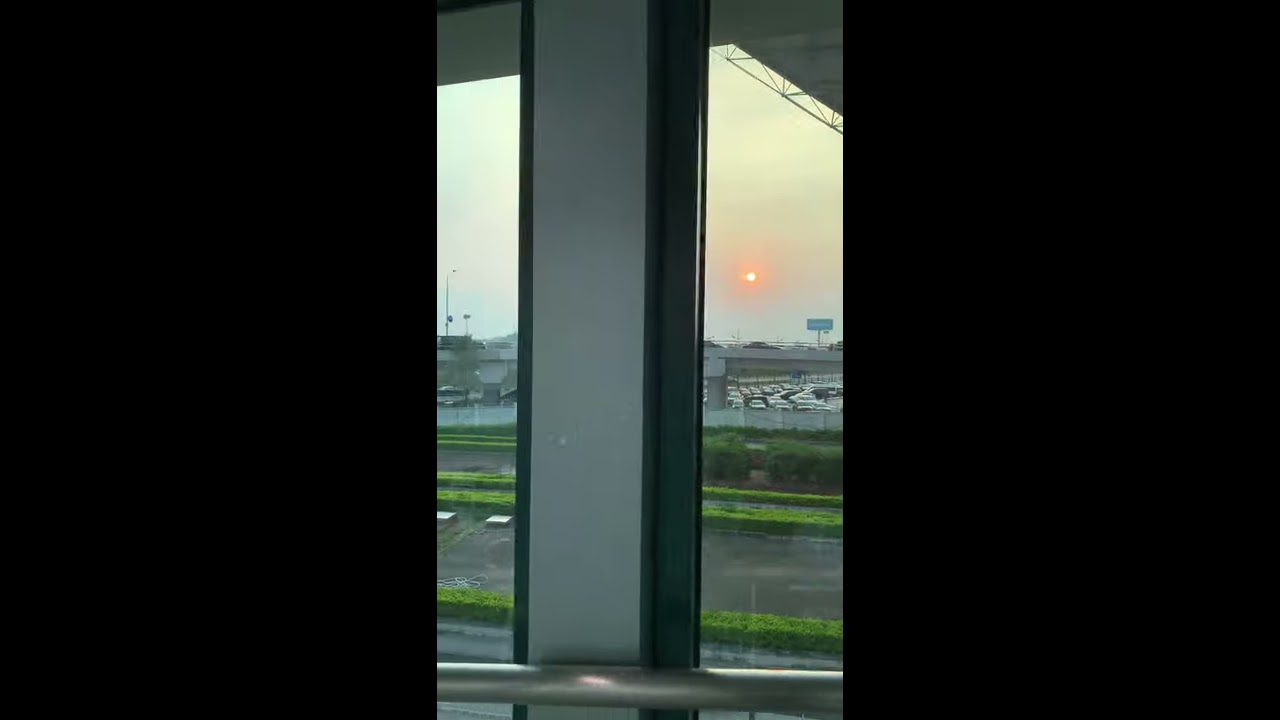The photo captures a scene framed by two silver-framed windows, with a central metal bar suggesting a possible railing or structural beam. Through the windows, the view reveals a well-manicured outdoor area featuring multiple rows of green, trimmed hedges leading toward a paved expanse. Beyond this foreground, a parking lot with scattered cars is visible, with a road or highway bridge stretching across the background. The setting sun, a deep orange disk with a white center, casts a warm hue over the scene, blending with the hazy, blue-white sky. In the distance, there are rolling hills or mountains, enhancing the picturesque backdrop. The very top of the image hints at the building's overhang, indicating the perspective is from indoors looking out.